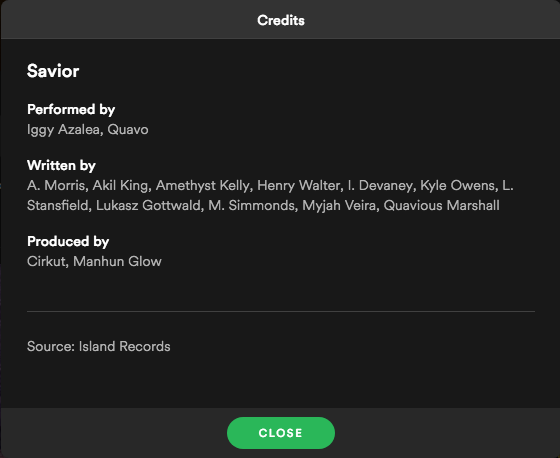The image showcases a credits screen with a black background and a dark grey foreground highlight, labeled "Credits." It provides detailed information about the song "Savior" performed by Iggy Azalea and Quavo. The songwriting credits include A. Morris, Akil King, Amethyst Kelly, Henry Walter, L. Devaney, Kyla Owens, L. Stansfield, Lucas Gottwald, M. Simmons, Maya Vieira, and Quavious Marshall. The track is produced by Circuit and Manhunt Globe and is released under Island Records. The layout appears to be reminiscent of a music streaming platform, possibly Spotify. At the bottom of the credits box, there is a "Close" option available for users to exit the screen.